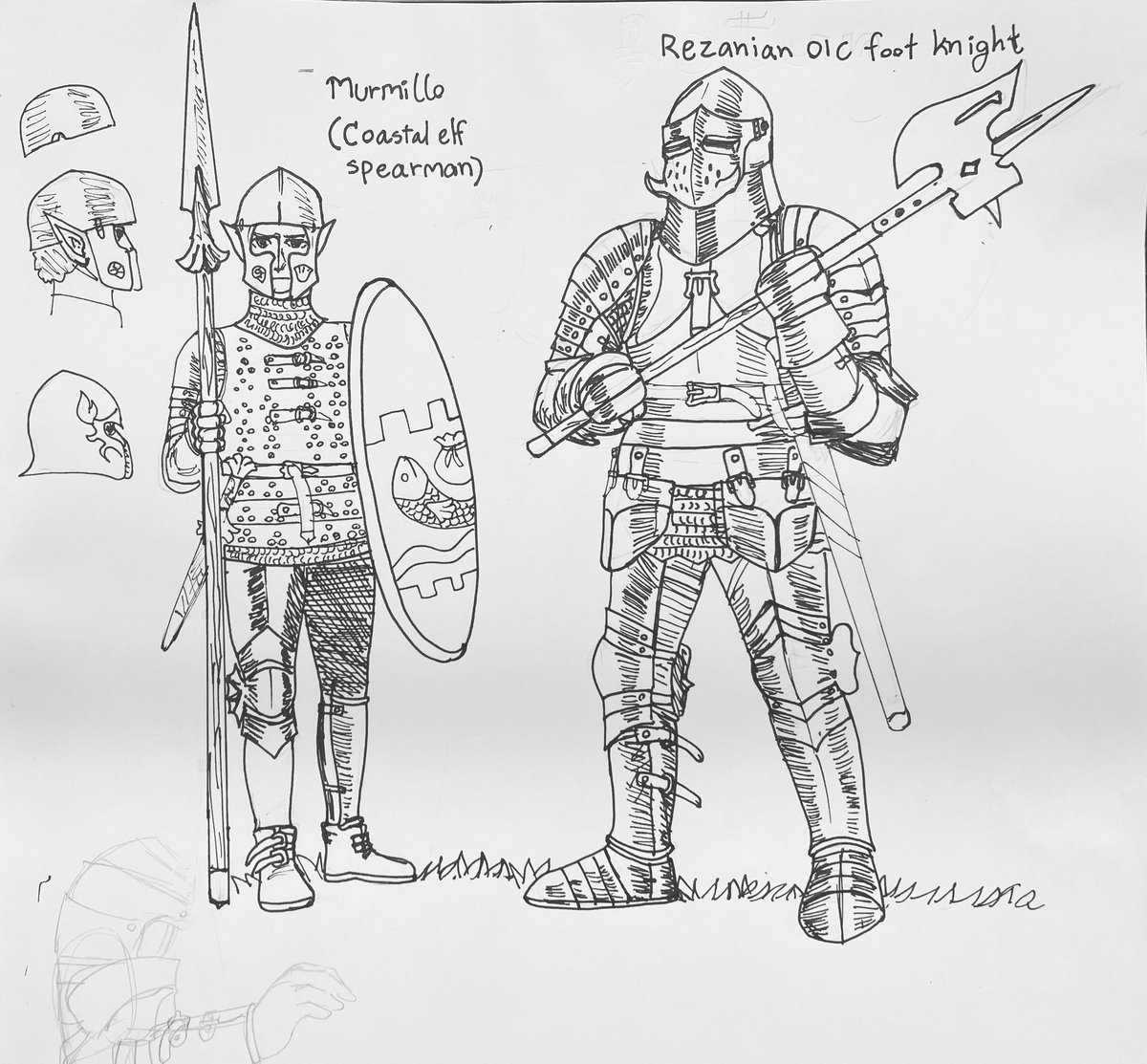This detailed pencil drawing features two knights prominently positioned on the left side of the artwork. The smaller knight on the left, identified by some as a "Murmillo" or coastal elf spearman, has distinctive elf ears and is clad in medium armor. He carries a large pointed spear with a wooden handle and an oval shield adorned with a fish emblem. Above him, pencil writing offers additional descriptions. The larger knight on the right, referred to as a "Wazanian oak foot knight," towers over his companion, wearing full heavy armor that encapsulates his imposing stature. He wields a massive war axe with a wooden handle, his name inscribed above. Both knights stand on a lightly sketched bed of grass. Surrounding these central figures are detailed studies and rough drafts, including a helmet diagram illustrating the top cap, face guard, and leather overlay, as well as a faint sketch of an arm in a metal sleeve in the bottom left corner.